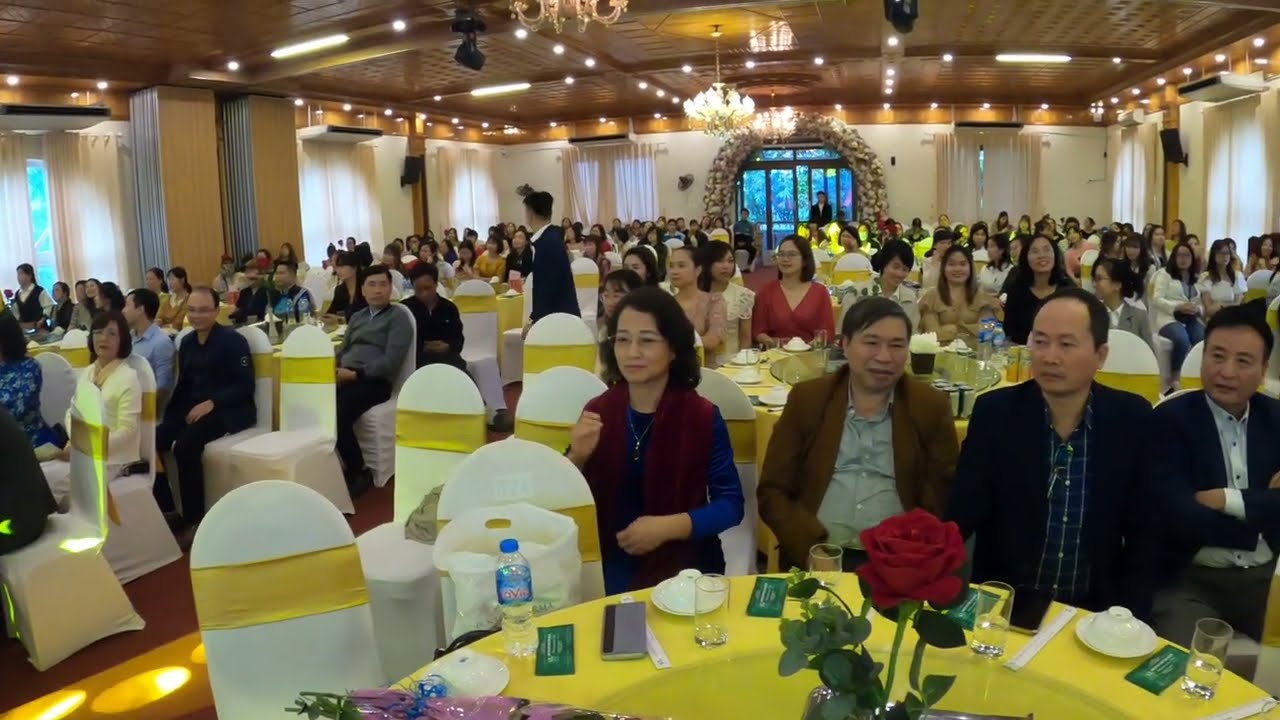In a grand, expansive banquet hall with high ceilings and elegant chandeliers, a formal event, likely a wedding reception, is in full swing. The room is adorned with ornate decorations, including large white curtains on the windows and intricate designs around the double glass doors at the far end. The tables, covered with vibrant yellow tablecloths, are neatly arranged with white chairs, each tied with a matching yellow band. At the center of each table sits a vase with a red rose, surrounded by plates and glasses. The atmosphere is lively and sophisticated, with over a hundred guests, mostly Asian, dressed formally in dresses and jackets. The majority of the guests are facing the front of the room, possibly towards a stage or a focal point of the evening's festivities.